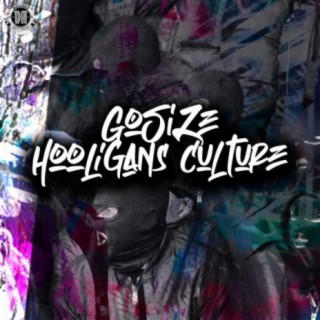The image is a small, square advertisement featuring intricate, abstract graphic design elements. In the center, white, fancy graffiti-style text reads "Go Size" on the first line and "Hooligans Culture" on the second line, albeit with some portions of the letters missing. The lettering also has a unique feature where each consonant has a small line underneath it. The background is a mix of graffiti art and abstract visuals, including elements like close-ups of tree trunks, sunlit areas, and colors that transition from gray to purple and blue. On the right side, there are figures wearing hoods and masks, dressed in gray clothing, adding a mysterious, urban vibe to the image. The top left corner features a black circle with "Da" in gray and a gray crown above it. The overall composition suggests a blend of natural and urban environments, creating a dynamic, provocative visual that is both eye-catching and enigmatic.